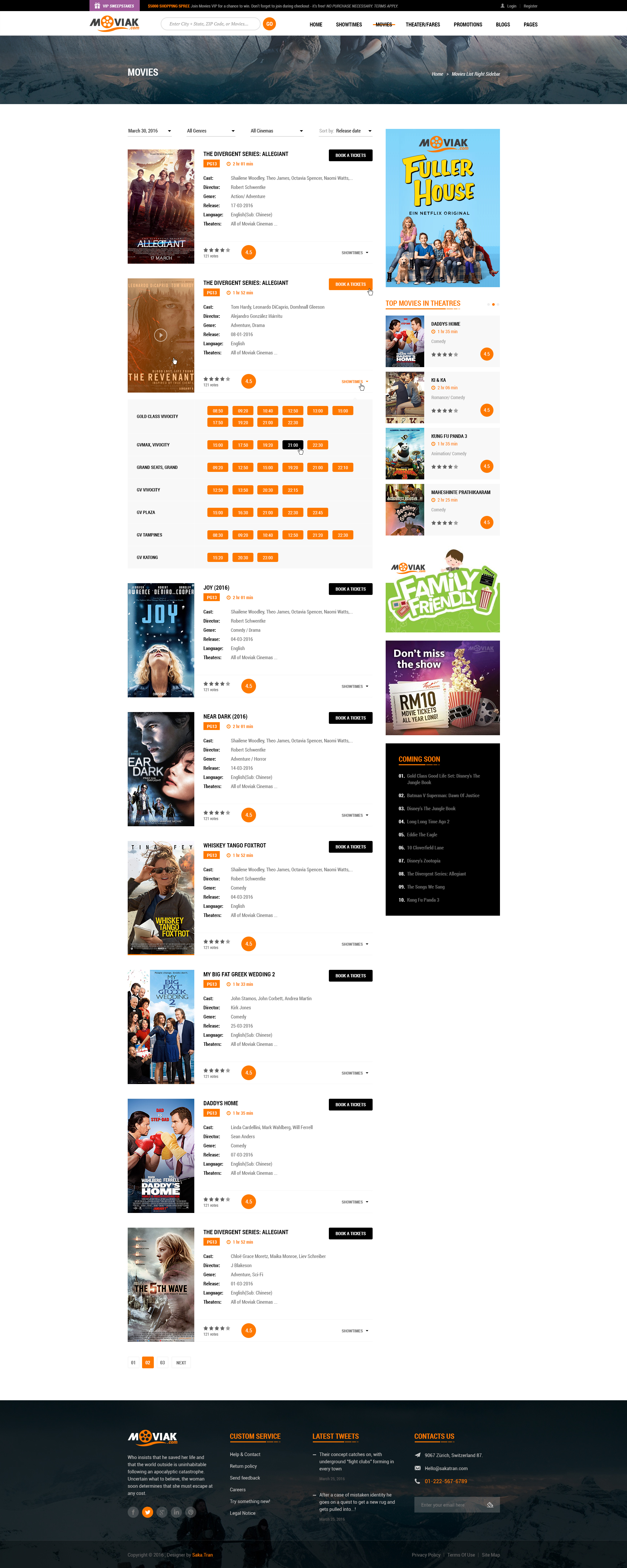The image depicts a screenshot from the website moviac.com, albeit significantly zoomed out and requiring close inspection to discern the details. Upon zooming in, the website’s layout and key functions become visible. 

At the top of the page, there is a search bar prompting users to "Enter City, State, Zip Code, or Movies" accompanied by a "Go" button. The main navigation menu includes options labeled as Home, Showtimes, Movies, Theater/Fairs, Promotions, Blogs, and Pages, with the "Movies" section currently selected. The date displayed is March 30th, 2016.

In a section labeled "All Genres," sorted by release date, the list begins with the movie "Allegiant" from the Divergent series, rated PG-13, with a runtime of two hours and one minute. The option to "Book A Tickets" is prominently displayed, along with additional details such as Cast, Director, Genre, Release Date, Language, and Theaters.

To the right, there is a banner featuring the logo and URL of moviac.com, alongside an advertisement for the Netflix Original series "Fuller House." 

Beneath this banner is an image promoting the movie "The Revenant," where a "Book Tickets" button is highlighted, revealing a dropdown menu with various seating options available for purchase.